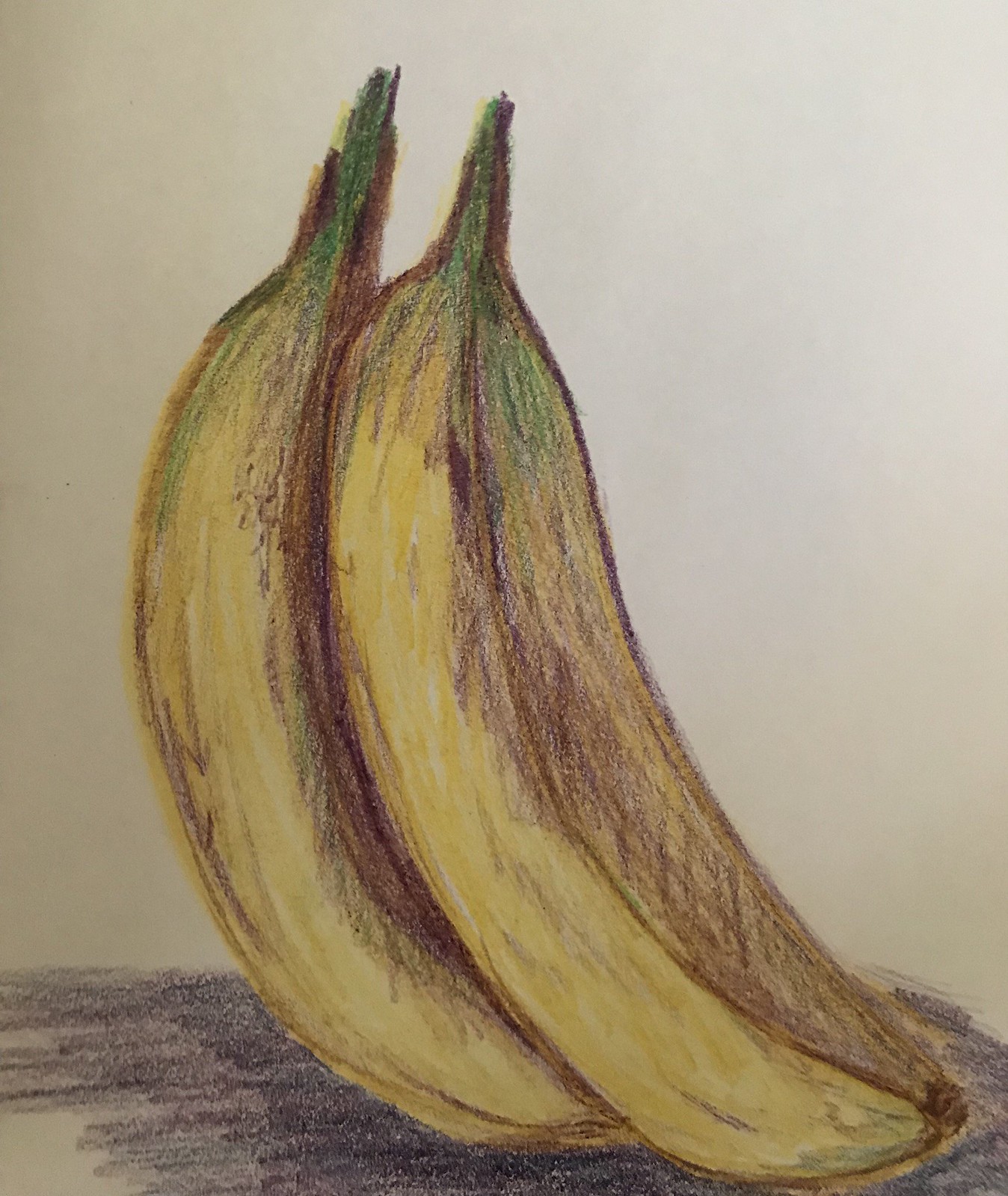This is a meticulously crafted colored pencil drawing of two bananas, rendered on an off-white sheet of paper. The bananas rest on a dark, undefined surface, creating a striking contrast that highlights their detailed textures and colors. The front banana is fully visible, showcasing a rich yellow hue along the bottom, gradually transitioning to a brownish tone towards the top. Its green stem is prominently displayed, while the tip is accented with brown spots. The second banana, partially obscured by the first, mimics these details, with only its lower portion visible. Intricate shading in shades of brown, white, and green further enhances the realism of the bananas, giving them a nuanced, lifelike appearance.